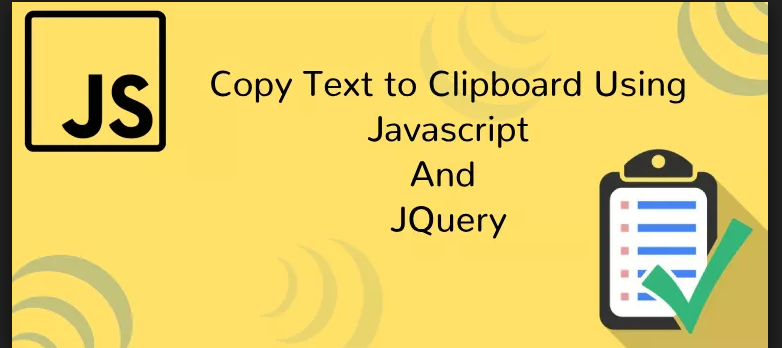This image features instructions flanked by thin black bars running vertically along both the left and right edges. The central background is a solid yellow, adorned with semi-circular patterns resembling Wi-Fi symbols in alternating dark grey and light grey hues positioned in the upper left corner. Prominently located in this corner is a square with thick black borders, its interior filled with the same yellow color as the background. Occupying the entire bottom quarter within this square are the bold, capital initials 'J' and 'S'.

At the center of the image, there is a text instruction that reads, "Copy text to clipboard using JavaScript and jQuery." Towards the bottom right, a black illustration of a clipboard holding a white piece of paper is depicted. This paper is marked with five orange bullet points, each paired with a blue line representing a list item. Extending from the bottom of the clipboard and overlapping the yellow background is a large green checkmark, symbolizing the completion of the task.